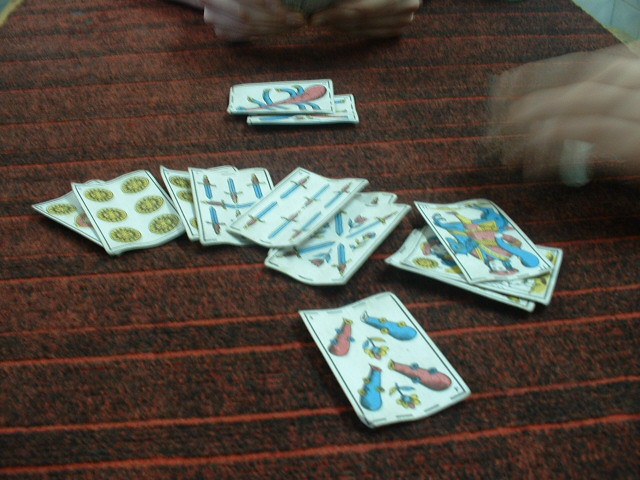The photograph depicts an intense card game in progress. The playing surface is characterized by a reddish-black color, featuring intricate red lines forming patterns across it—thin red lines alternate with varied spaces, creating a visually striking grid. In the foreground, two pairs of hands are visible. On the far side, only the edges of the players' hands are seen. On the left-hand side of the image, the right-hand player’s hand appears blurred, suggesting rapid movement, and possibly adorned with a white ring on the pinky finger.

Scattered across the table are multiple cards, some displaying vibrant blue and red designs. Among them, three cards appear to have joker illustrations, while another stack of cards showcases images of six yellow coins. Additionally, some cards depict knives arranged in various formations—some with six knives positioned vertically and horizontally, others forming an X shape interspersed with floral designs. This detailed arrangement of cards provides a rich visual narrative, capturing the strategic and dynamic atmosphere of the game.